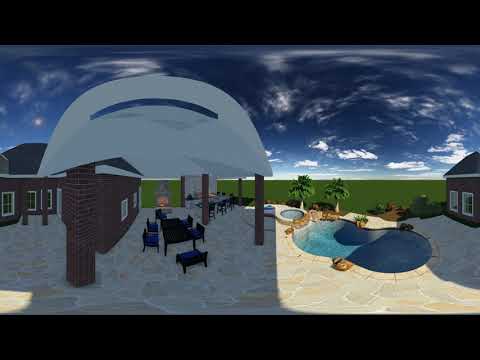This detailed image, possibly a digitally created scene for a video game or television screen, depicts an outdoor area combining elements of a beach house setting. The photograph is cropped, showcasing both a sunlit and shadowed environment. The upper half of the image features a sky transitioning from navy blue to a lighter blue closer to the horizon, dotted with white clouds.

In the foreground, on the right side, there's an inviting in-ground swimming pool accompanied by a sauna or hot tub at its corner. The pool area has a cement deck complete with a table and chairs, which are adorned with blue cushions. Adjacent to the pool, a brown brick building stands next to a table with a white awning. This side reveals more of the patio, including the sunny and grassy sections with a couple of palm trees.

On the left side, in shadow, more of the brick house is visible, highlighting additional doorways and an outdoor courtyard area, as well as an outdoor fireplace. The entire scene suggests a contrast between two environments, enhanced by the depiction of both sunny and possibly snowy weather conditions, hinting at different seasonal settings or perhaps different geographical locations like Palm Beach, Florida, or Palm Springs, California. There's an outdoor table and chairs set on this side as well, similarly equipped with blue cushions, emphasizing the area's cozy, yet tropical ambiance.